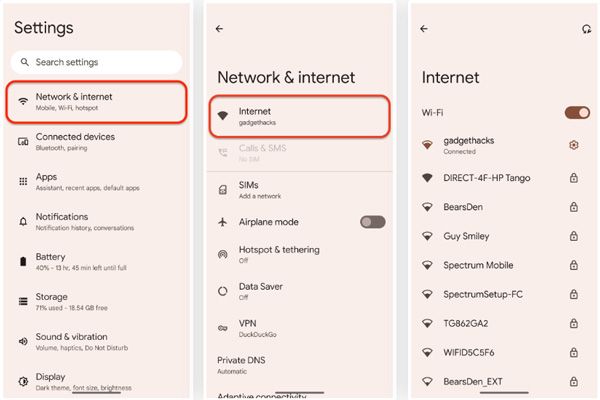A series of screenshots displayed against a peach background details the navigation through device settings. The first screenshot features the "Settings" menu, highlighted by a red rectangle around the "Network & internet" option. Below the highlighted section, various settings options are visible including "Connected devices," "Apps," "Notifications," "Battery," "Storage," "Sound," and "Display." The second screenshot shows the opened "Network & internet" menu, where an "Internet" icon is prominent at the top. Additional network options such as "SMS," "Airplane mode," "Hotspot," "Data," "VPN," and "Private DNS" are listed below. The third screenshot reveals an "Internet" submenu, displaying the current Wi-Fi status and a list of connected devices. Text across all images appears in black, providing clear labeling for each function and option.